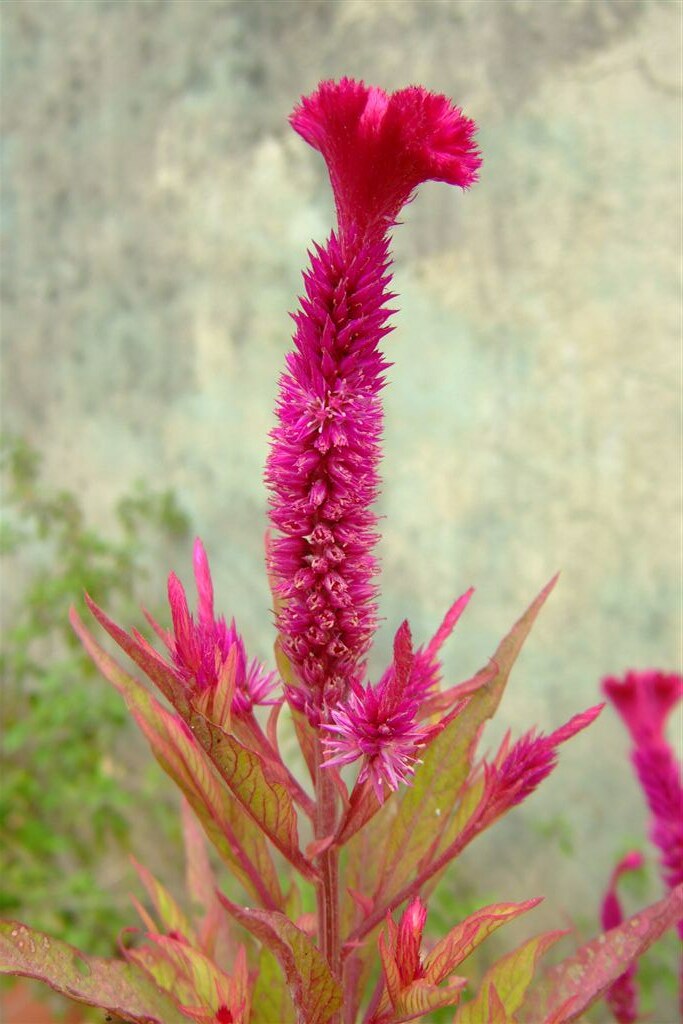This vivid photograph captures a striking tropical flower, showcasing its brilliant, almost neon, pinkish color. The flower, shaped like a long, narrow oval or cone, begins with a spiky middle section that transitions into soft, silky blossoms at the top. The green leaves, which have pink-purplish veins running through them, complement the vibrant hue of the flower. In the bottom right corner, another similar flower is visible, further emphasizing the plant's exquisite beauty. To the bottom left, there are blurry green leaves from another plant, recognizable only by their shape. The distant background is a hazy blend of light green and brown, potentially depicting more foliage or a wall, adding to the natural ambiance and suggesting an outdoor setting. The image also includes smaller buds in the same vibrant pink and additional elongated flowers in the background, enhancing the lush, tropical feel.